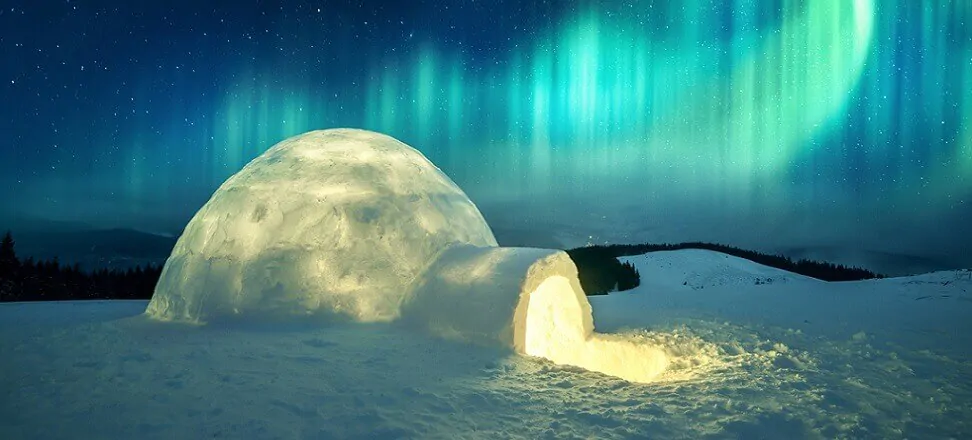The photograph captures a serene nighttime winter scene featuring a glowing igloo in the foreground, slightly to the left of the center of the image. The igloo has a dome-shaped, hemispherical structure with a small, rounded entrance pointing towards the lower right. Illuminated from within, the igloo emits a gentle white to light yellow glow, which is most pronounced at the entrance. Surrounding the igloo is a snow-covered field, extending across the entire scene from left to right. Behind the igloo, there is a subtle line of trees, primarily evergreen, which run horizontally across the distant horizon, with rolling hills visible in the background.

Dominating the upper half of the image is a captivating sky filled with the northern lights, or aurora borealis. These vertical swaths of greenish and lighter blue light traverse the dark blue sky, enhancing its vibrant, celestial beauty. The sky is peppered with numerous stars, adding to the overall ethereal atmosphere of the scene. The combination of the glowing igloo, the dark trees, and the striking northern lights render this photograph a magical representation of an Arctic landscape.